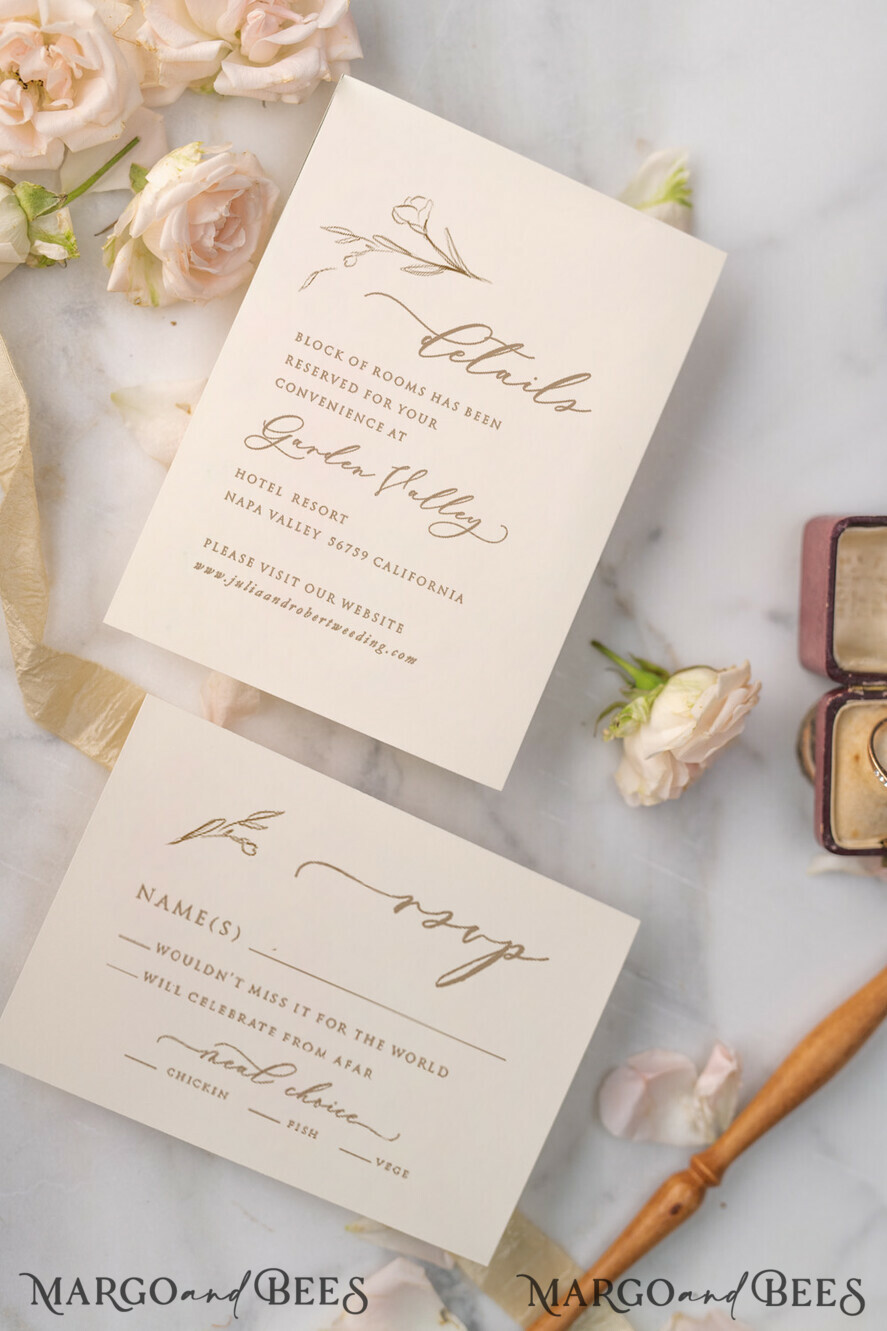The photograph capture shows a set of elegant stationery arranged artfully against a sophisticated backdrop. Two cream-colored, rectangular cards are tilted 45 degrees to the right. The top card, approximately the size of a standard 8 by 10 sheet, features detailed event information in a sophisticated golden script, mentioning a reserved block of rooms at Napa Valley's Garden Valley Hotel Resort, and provides a website for further details. The bottom, slightly wider, card is an RSVP response card with options for attending or celebrating from afar, along with meal choices such as chicken, fish, or vegetable. Both cards are embossed in pale brown, luxurious lettering.

A watermark at the bottom displays "Margot and Bees," suggesting the brand of the high-end stationary. The background is a chic white marble, accented by delicate, faux pale pink roses with green stems scattered at the top, right side, and petals at the bottom. A wooden utensil forms a triangle at the bottom of the arrangement, adding a rustic touch to the elegant display. This intricate composition highlights a blend of luxury and meticulous craft, making the stationary stand out prominently.